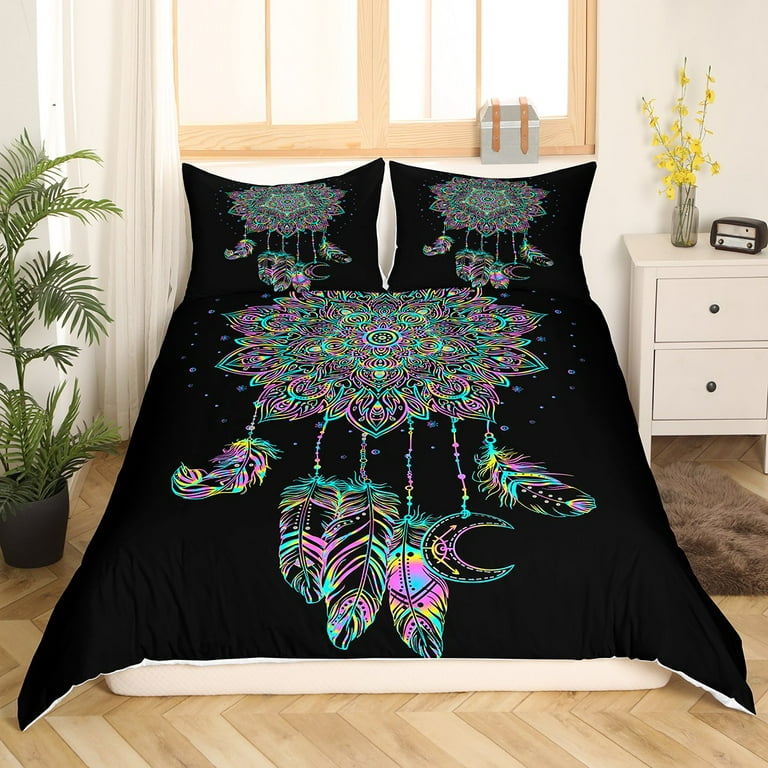This image features a bedroom with a centrally positioned bed, viewed from the front. The bed is dressed in a striking black bedspread, including both the comforter and pillows. The comforter and pillows showcase an intricate, colorful pattern featuring light blue, pink, yellow, and black. The lower part of the white mattress is visible beneath the bedspread. 

The room's flooring is a light brown shade, adding warmth to the space. Positioned to the left of the bed is a tall house plant, standing in a sleek black pot. The plant has blade-like leaves that extend upwards, reaching about two to three feet, slightly surpassing the height of the bed.

On the right-hand side, a white end table with two drawers adorned with black knobs is placed against the wall. Atop the end table sits a small vase filled with vibrant yellow flowers and a black alarm clock. Above the table, the lower part of a lightly brown window frame is visible, completing the cozy and aesthetically pleasing bedroom setup.